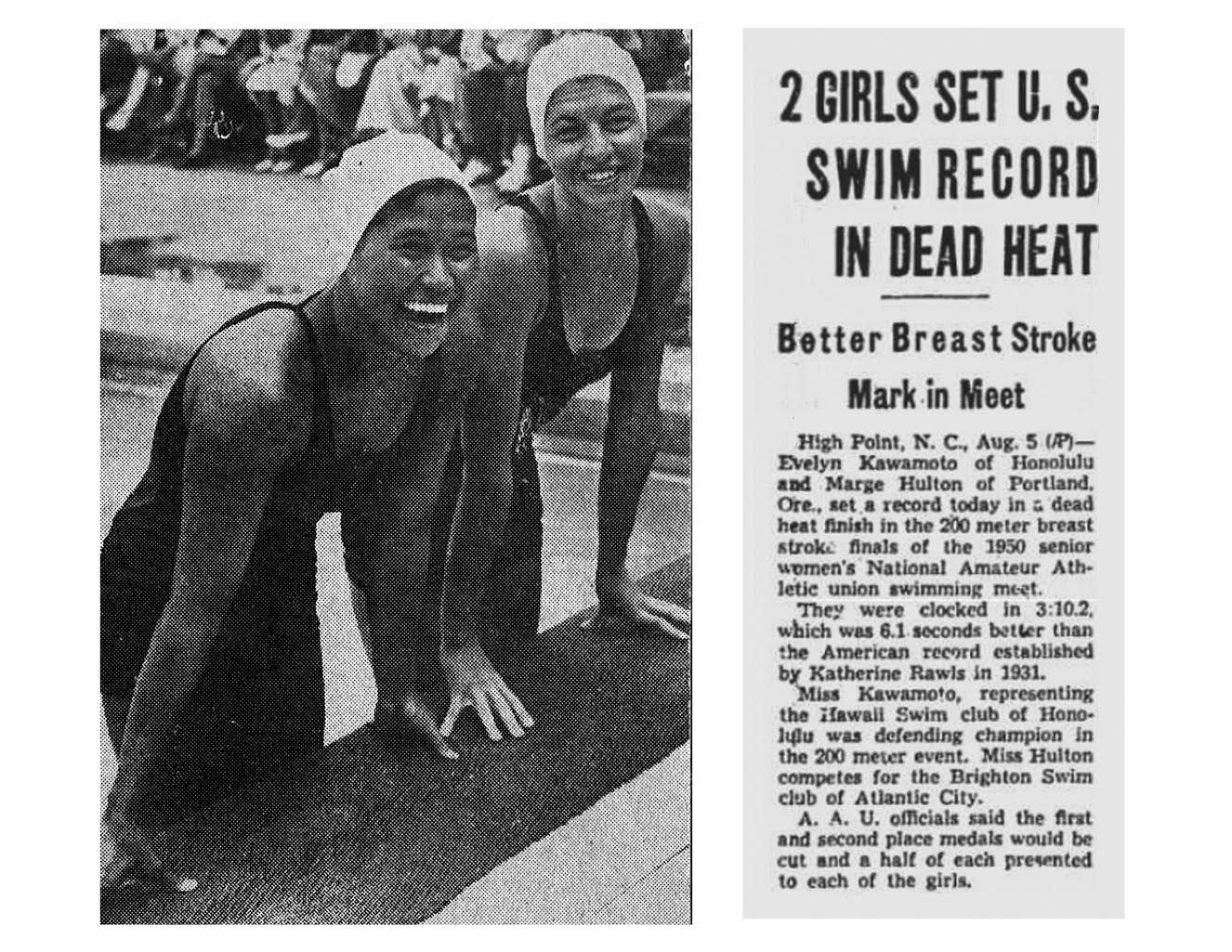This is a black and white newspaper clipping featuring an image and an article about a remarkable achievement in swimming. The photograph, positioned on the left, captures two female swimmers, Evelyn Kawamoto of Honolulu and Marge Halton of Portland, Oregon. They are seen partially submerged in a pool, smiling broadly at the camera while propping themselves up on the edge of the pool with their hands. Both women are wearing dark, one-piece swimsuits and white swim caps.

In the background, there are rows of benches filled with spectators, indicating that this event took place outdoors. The accompanying article headline, "Two Girls Set U.S. Swim Record in Dead Heat," is prominently displayed. It provides details of their record-setting performance in the 200-meter breaststroke final at the 1950 Senior Women's National Amateur Athletic Union (AAU) swimming meet in High Point, North Carolina. 

The article celebrates their achievement, noting that they clocked in at an impressive 3 minutes and 10.2 seconds, surpassing the previous American record held by Catherine Rawls since 1931 by 6.1 seconds. It further mentions that Evelyn Kawamoto was the defending champion, representing the Hawaii Swim Club of Honolulu, while Marge Halton competed for the Brighton Swim Club of Atlantic City.

A unique aspect of their win was the decision by AAU officials to split the first and second place medals in half, with each swimmer receiving a segment, reflecting their tie. The typeface and quality of the photograph suggest the article's vintage origin from the 1950s.